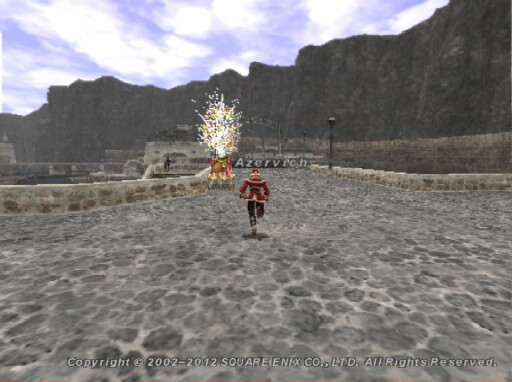A vibrant screenshot from a video game, possibly created by Square Enix Co., Ltd. as indicated by the copyright text "2002-2012 Square Enix Co., Ltd. All Rights Reserved" at the bottom. The scene captures a wide, gray stone walkway flanked by a short, approximately three-foot-high stone wall on one side. At the center of the walkway, a stylized, cartoon-like character is seen in mid-run, adorned in a striking red and gold jacket paired with black pants. In the distant background, a dramatic yellow and white explosion creates a dynamic and intense atmosphere, suggesting a high-stakes moment in the game.